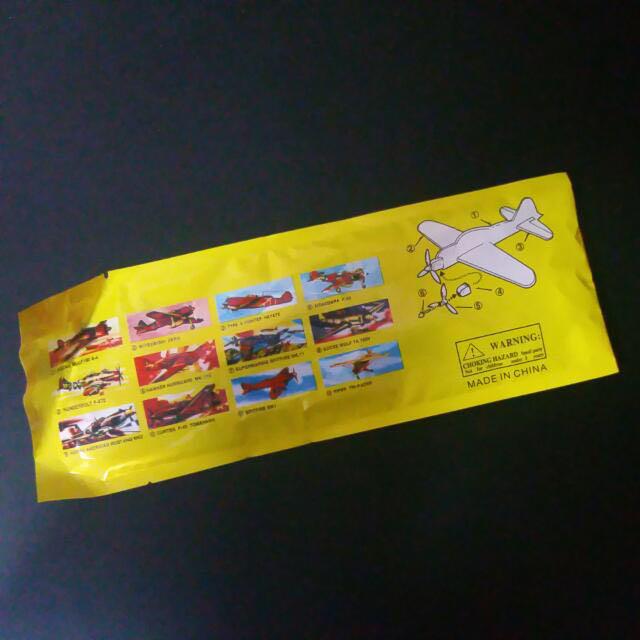This image features a yellow wrapper, likely for a wooden self-assembly model airplane toy, set against a black background. The package is displayed backside up, obscuring the name of the toy. Prominently featured on the left side is a four-by-three grid, showcasing twelve photographs or mockups of vintage WWII airplanes, predominantly red and red-and-white. Adjacent to this grid, on the right side of the wrapper, is a white diagram illustrating the assembly process of the toy, specifically highlighting the placement of the propeller. Below this diagram, a rectangular warning box plainly states a choking hazard. Further below, in all capital letters, is the text "MADE IN CHINA." The wrapping material appears to have tear-indentation marks along the top and bottom edges.